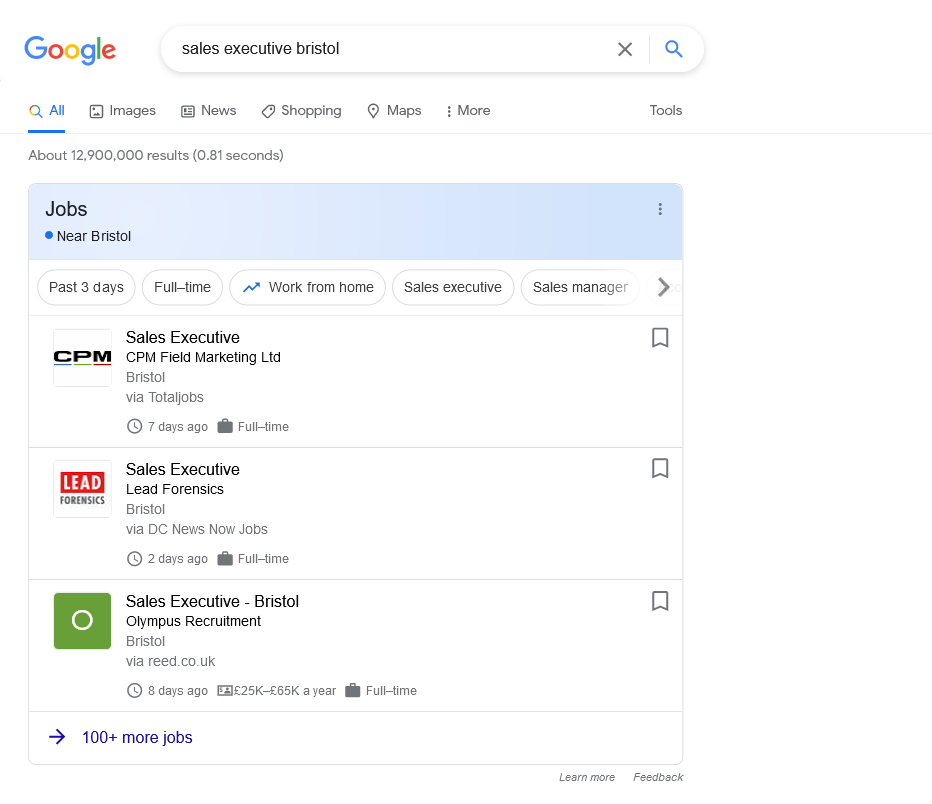A screenshot captured on a tablet device, most likely an iPad, depicts a Google Jobs search for a "sales executive" within the Bristol area. At the top of the screenshot, the recognizable Google logo, featuring the colors blue, red, yellow, blue, green, and red, is displayed on a white background. The search term "sales executive Bristol" is visible in the search bar.

The interface showcases various tab options, including "All," "Images," "News," "Shopping," "Maps," "More," and "Tools." The search results indicate that approximately 12,900,000 results were found in 0.81 seconds. The page is filtered to show job listings available in the past three days, categorized under full-time positions, work from home options, sales executive roles, and sales manager roles.

Highlighted are three specific job listings in the Bristol area:
1. A Sales Executive position at CPM Field Marketing in Bristol.
2. A Sales Executive role at Lead Forensics in Bristol, listed as a full-time job and posted two days ago.
3. A Sales Executive opportunity with Bristol Olympus Recruitment, also a full-time position, posted one day ago.

This comprehensive overview provides a detailed portrayal of the job search snapshot, emphasizing the various elements and search results visible in the Google Jobs interface.